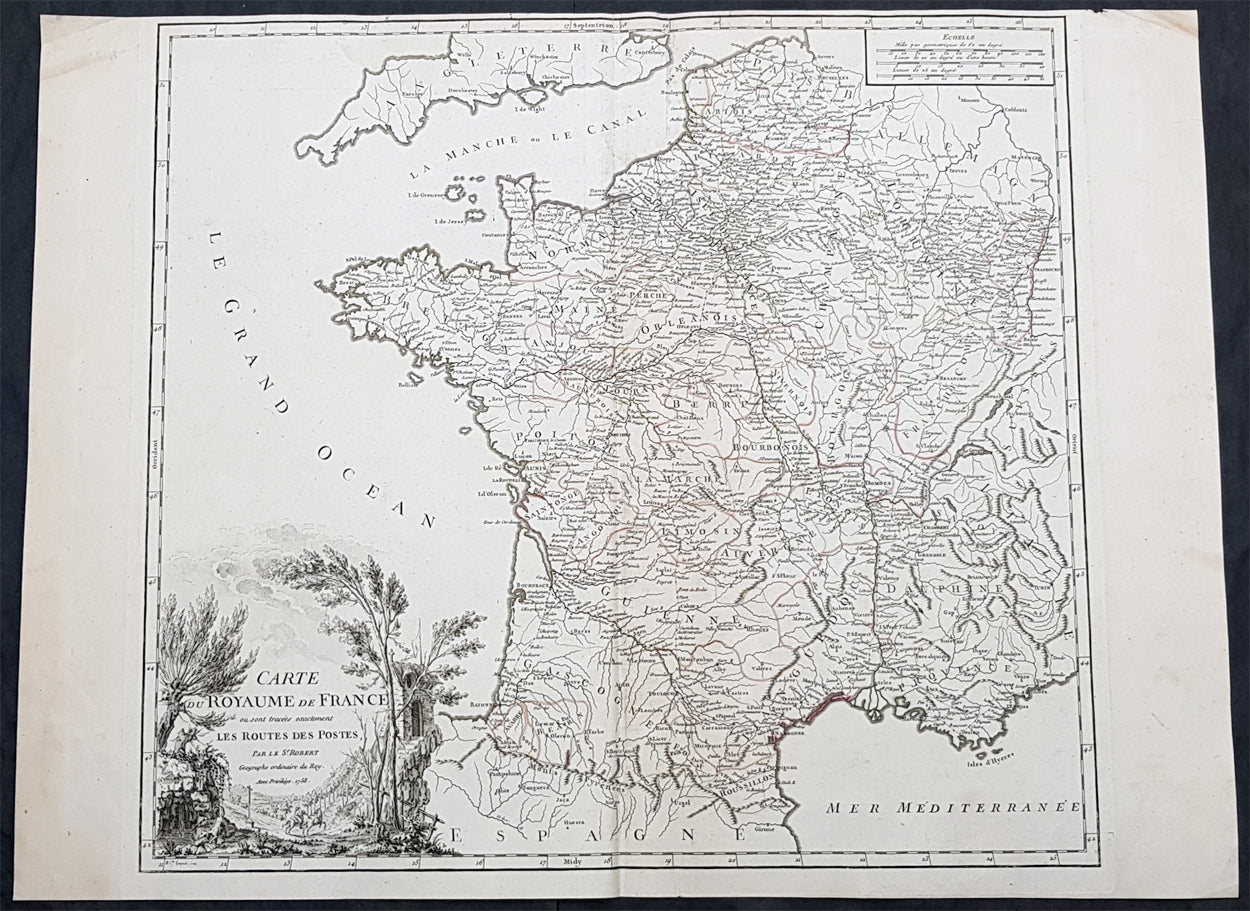This intricate, black-and-white drawn map on aged paper, possibly with water stains, depicts parts of Europe primarily labeled in French. The detailed map showcases Spain, France, and mentions La Grande Ocean along the left side and Mer Méditerranée to the right. The text "Carte Royaume de France" suggests it principally concerns France. The map includes minute, difficult-to-read lettering marking cities, canals, and rivers. In the upper left corner, a grid or scale is visible, while the lower right corner features illustrations of a forest scene with possibly trees, a building, and a horse, indicative of the map's artistic nature. Despite its small and blurred text, the map's detailed routes and geographic information hint at its historical and educational value.